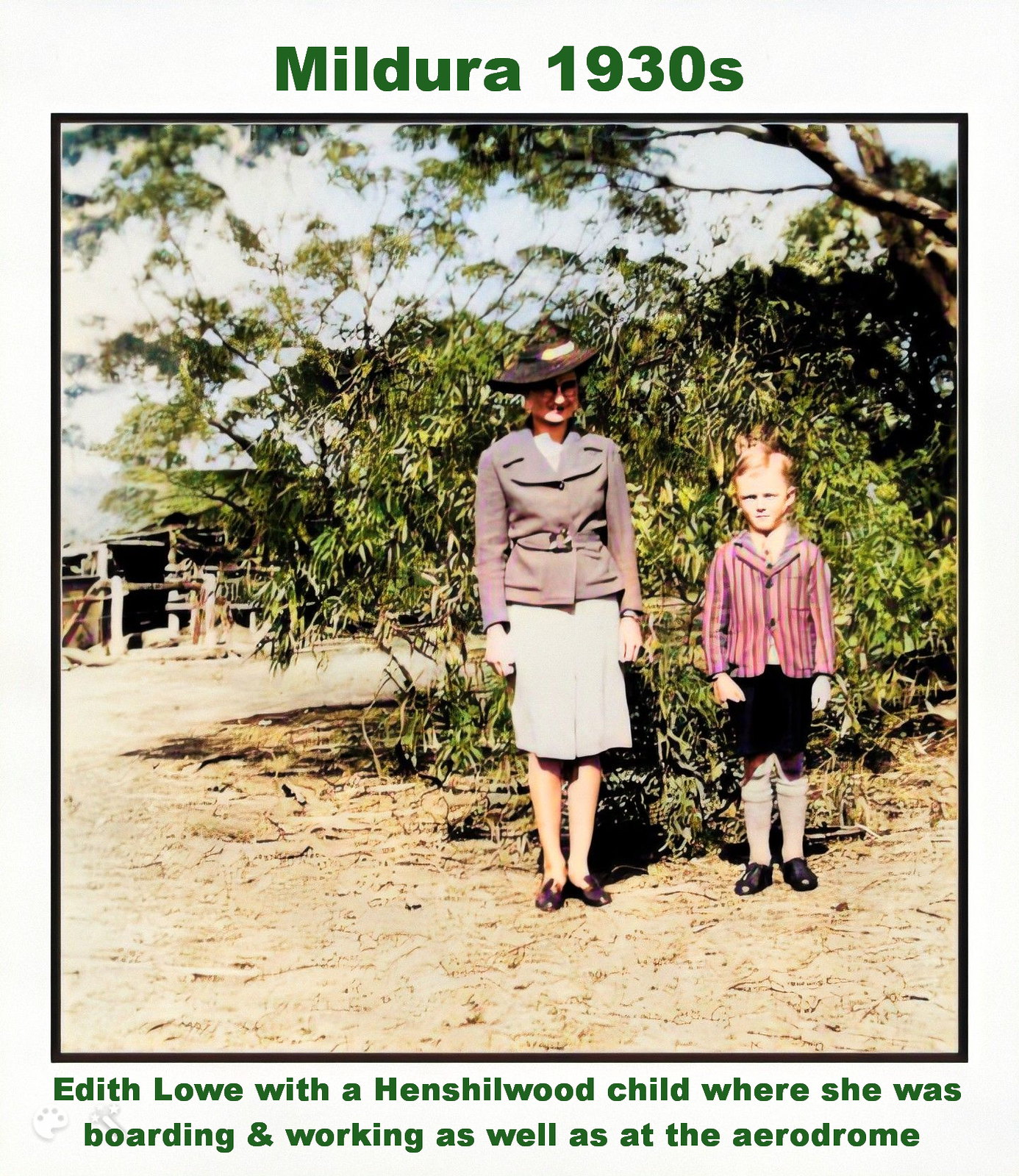**Mildura 1930s: Edith Lowe with a Henshelwood Child**

This vintage photograph, enhanced with hand color tinting, presents a poignant slice of life from the 1930s. The photograph features an older woman, identified as Edith Lowe, standing centrally and looking toward the viewer. Edith is dressed in a sophisticated attire, including a large dark brown hat perched stylishly to the side, a brown suit jacket over a white dress that reaches her knees, and dark brown shoes. Accompanying her on the right is a young boy, the Henshelwood child, who is attired in a distinctive pink jacket with purple stripes, black shorts, tall white socks, and black shoes. The boy's reddish-brown hair is neatly side-parted as he gazes directly at the camera.

Set against an outdoor backdrop, the image captures a large tree and a hutch in the background, adding depth and context to the scene. The muted colors and the detailing provide a vivid contrast, highlighting the subjects against the natural environment. The photograph is bordered in a light gray background with dark green headings. At the top, "Mildura 1930s" is prominently displayed, while the subcaption underneath reads, "Edith Lowe with a Henshelwood child where she was boarding and working as well as at the aerodrome." The artistic combination of vintage photography and modern graphic design elements enhances the nostalgic yet timeless appeal of the image.